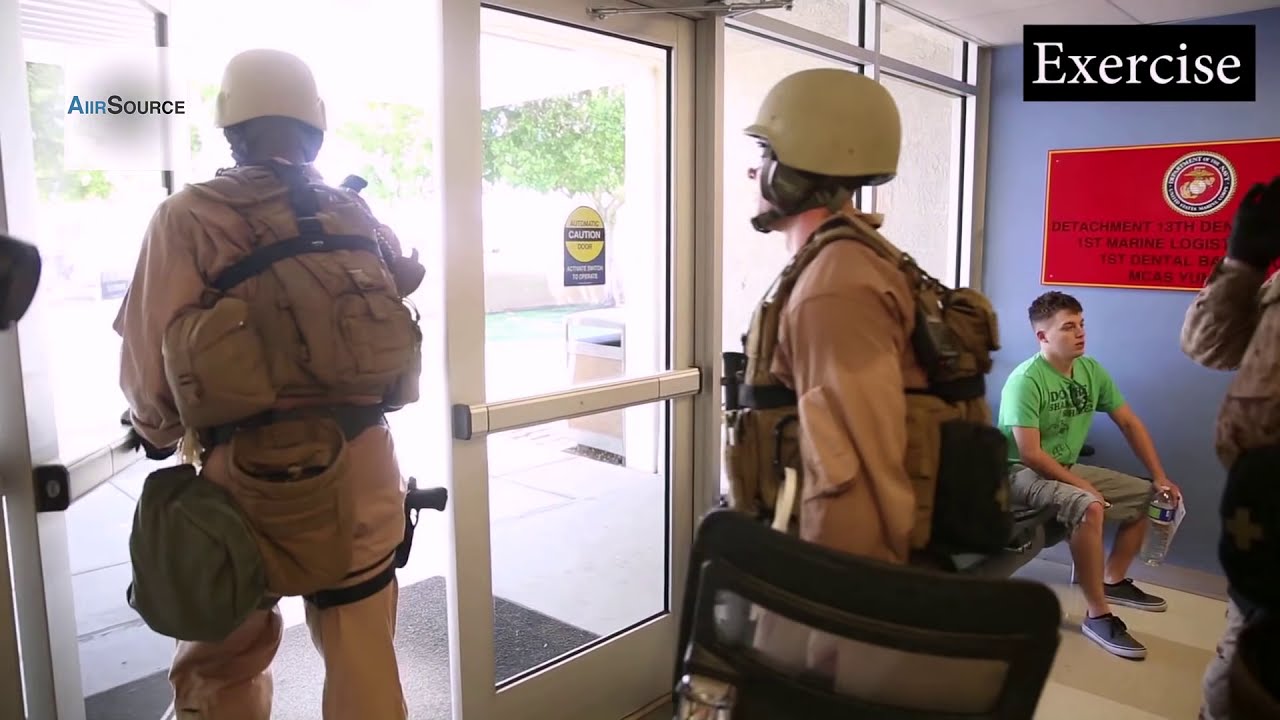In the image, two men, likely soldiers based on their tactical or military-style gear, are seen exiting a building through a doorway typical of a grocery store entrance. The man in the foreground holds the door open for the one behind him. Both are dressed in tan camouflage uniforms with dark green packs and possibly helmets, while the soldier on the left has a gun holstered on his right thigh. The soldier on the right might be holding a shield. Inside the building, a younger man, possibly a teenager around 15 to 17 years old, is seated on a bench against a blue wall. He is wearing a light green t-shirt with black lettering, khaki shorts, and dark shoes, looking away from the camera as if waiting for something. There is a partially visible red sign on the back wall that mentions "detachment 13th," "First Marine," and "First Dental," indicating a possible military setting. In the upper left corner of the image, text reads "Air Source" in blue and black, likely a logo, while the upper right corner features the word "exercise" in white text. The scenery outside the door suggests a sunny day with trees visible, possibly leading to a parking lot.